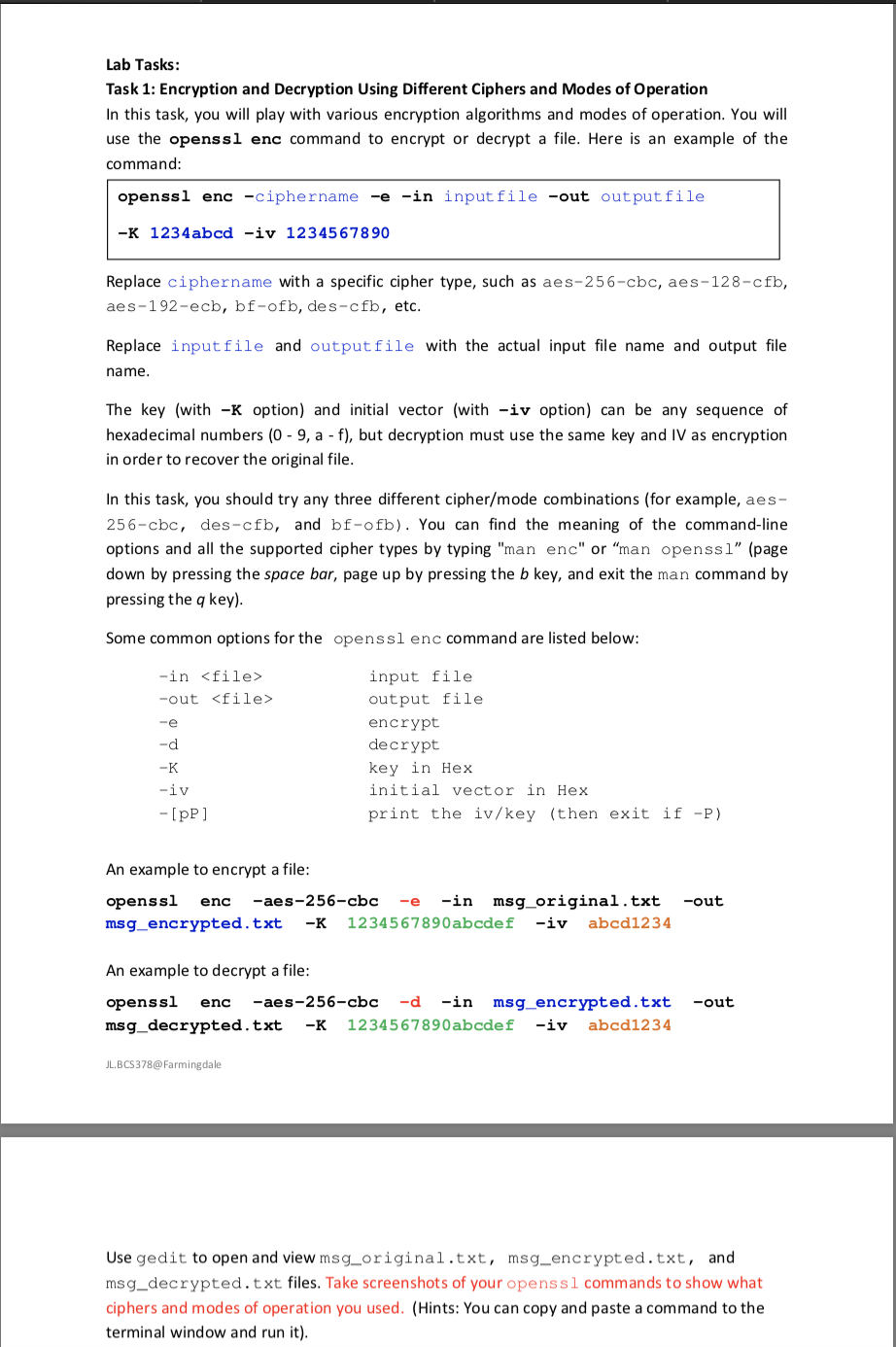### Detailed Caption:

This image showcases a page densely packed with text on a clean, white background, devoid of any photographs or drawings. The content begins by outlining "Lab Tasks," with "Task 1" focusing on "Encryption and Decryption using Different Ciphers and Modes of Operation."

In this task, users are instructed to experiment with various encryption algorithms and modes of operation using the `openssl enc` command for file encryption and decryption. A rectangular box on the page contains an example of the command, specifying placeholders such as `<cipher_name>`, which users should replace with specific cipher types. Examples of these types are listed within the text. Similarly, placeholders like `<input_file>` and `<output_file>` should be replaced with actual file names. Important details are provided about the key and initialization vector (IV): both must be sequences of hexadecimal numbers, and the same key and IV used for encryption must be reused for decryption to recover the original file.

The task requires participants to experiment with three different combinations of ciphers and modes, listing examples for each. To understand the `openssl enc` command and the variety of supported cipher types, users are directed to consult the manual pages (`man enc` or `man openssl`). Navigation instructions are provided: use the spacebar to move down one page, press 'B' to move up one page, and press 'q' to exit the manual.

The page details common options for the `openssl enc` command and provides explicit examples of both encryption and decryption commands. It instructs the user to use the text editor "gedit" to open and view files, listing specific file names for illustration. Lastly, users are advised to take screenshots of their results, showing the ciphers and modes of operation they employed throughout the task.